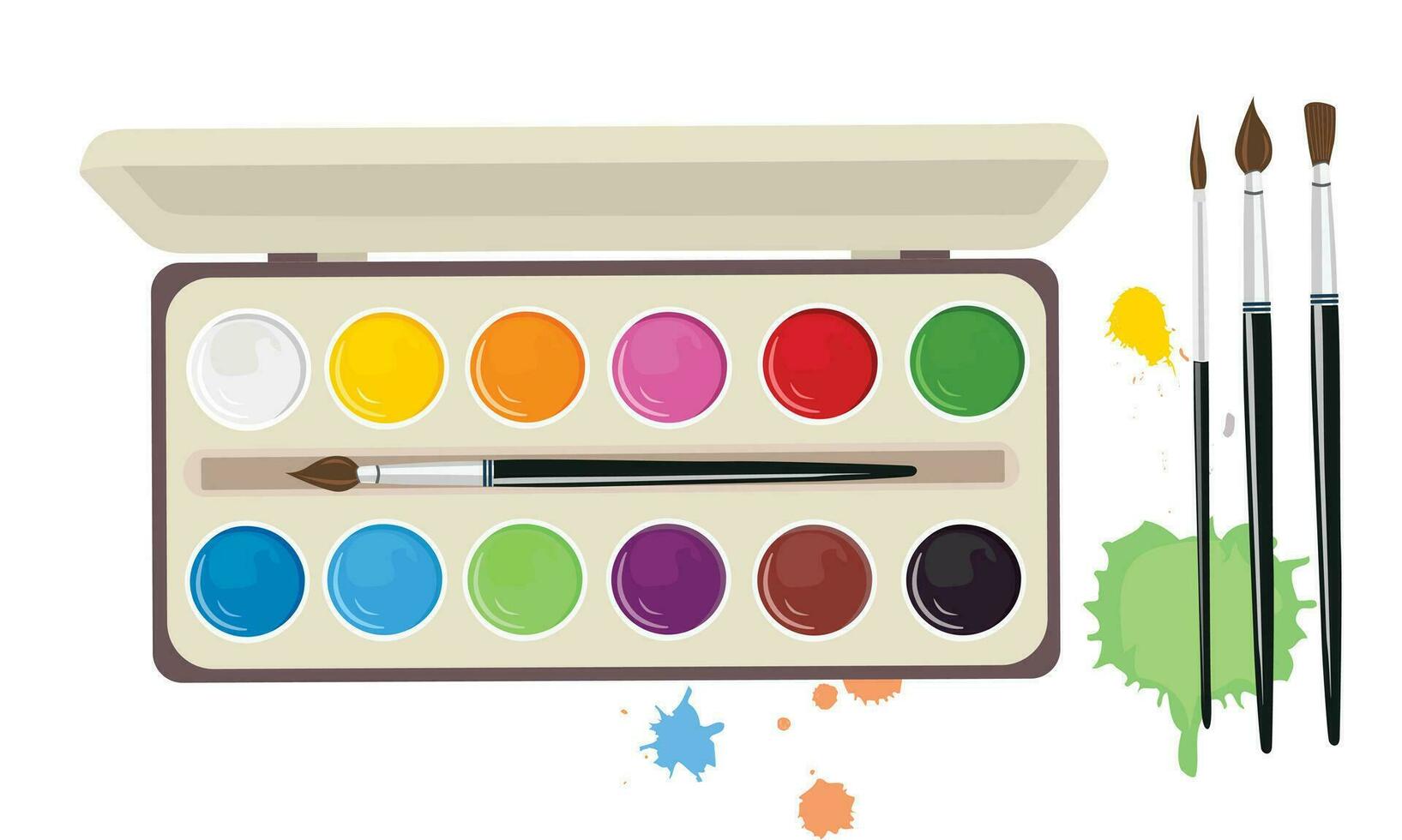This is an illustration of a watercolor paint set within a light gray, opened case with a darker gray border. The case showcases a neatly arranged display of twelve colors, starting with white, yellow, orange, pink, red, green, light blue, dark blue, lime green, dark purple, brown, and black. These colors are organized in two rows, six at the top and six at the bottom, with a paintbrush positioned horizontally across the middle of the palette. To the right of the palette, three vertically standing paint brushes vary in thickness, with handles that transition from black to white with blue lines, and dark brown tips. Scattered around the set are paint splotches: a large green splotch with a smaller yellow one above it, alongside other lighter-colored stains including maroon and blue. Overall, the illustration captures the vibrant and diverse tools essential for a watercolor artist.